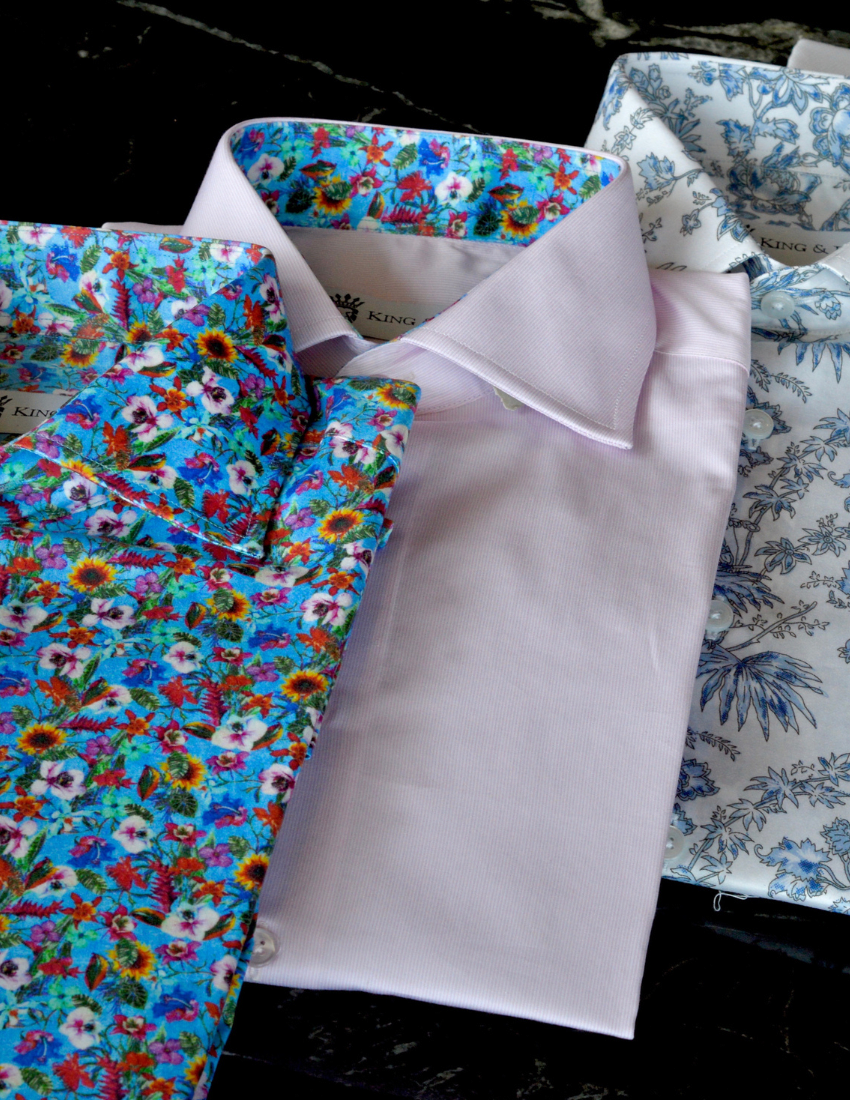The photo showcases three meticulously folded shirts, arranged diagonally from the bottom right to the top left, displayed on a sleek black marble surface with white veining. The shirts are stacked neatly with the first shirt on the bottom right. This shirt is a crisp white button-up with an intricate blue floral pattern. The center shirt, placed on top of the first, is a delicate light pink to almost purplish tone featuring thin stripes. Its collar reveals a hidden internal pattern of the same vibrant blue floral design seen on the shirt to its left. The topmost shirt, positioned to the left, is the most eye-catching with its dominant light blue color and a lively assortment of sunflower illustrations and small animals, primarily in yellow, red, orange, and green hues. All three shirts are labeled "King," though the full brand name is partly obscured by their collars.